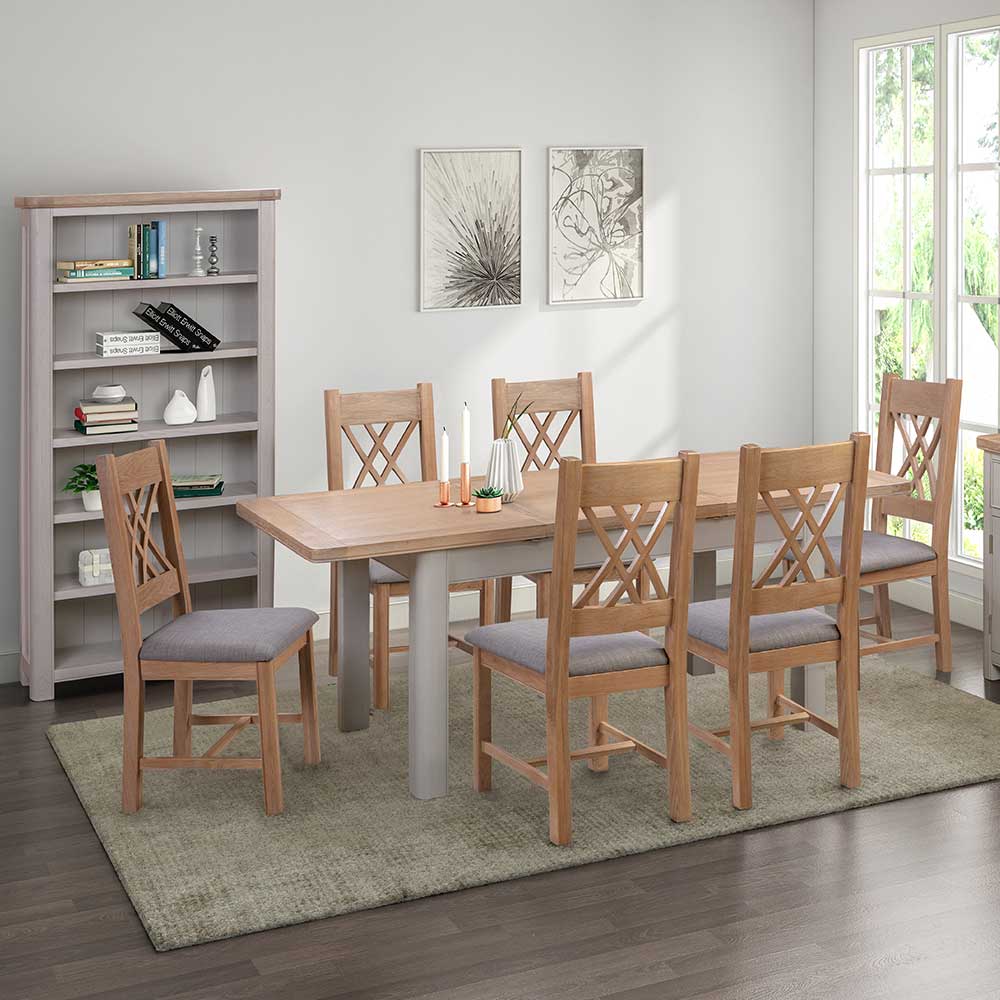The photograph captures a dining area inside a house with a minimal design theme. The room features white walls and polished hardwood floors. A vertical, rectangular wooden table with a brown top and gray legs is the focal point, accompanied by six wooden chairs with gray cushions and lattice-patterned backs. The table is positioned on a light brown area rug. To the right, tall double doors, likely leading to a patio, offer a glimpse of greenery outside. On the wall directly behind the table, there are two black-and-white framed artworks; the left one features a burst design, while the right one is abstract. Adjacent to the paintings, on the left, stands a gray bookcase stocked with books and a vase. The scene is completed by the natural light flooding in through the doors, enhancing the serene, minimalistic ambiance.